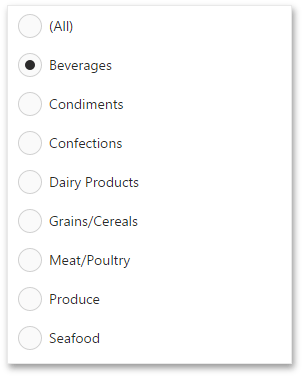This image features a white rectangle framed with a light blue border. Inside the rectangle is a vertical list of categories, each preceded by a circular checkbox that can be filled in. At the top of the list, "All" is written in parentheses. Following this, "Beverages" is listed, and its corresponding checkbox is shaded, indicating selection. The list continues with "Condiments," "Confections," "Dairy Products," "Grains/Cereals," "Meat/Poultry," "Produce," and "Seafood," all of which have empty checkboxes. The graphic is devoid of any additional markings or illustrations.